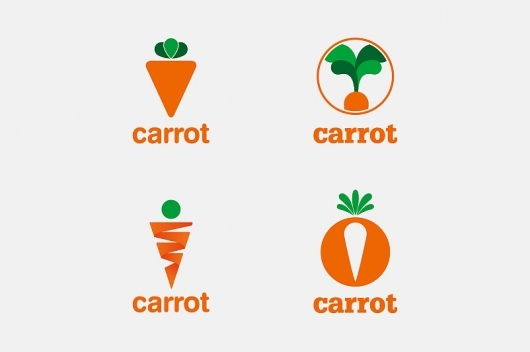This image showcases a collection of four carrot-themed logos on a white background, arranged in a 2x2 grid, each with the word "carrot" beneath them. The logos are designed in orange and green, utilizing different styles to represent carrots:

- The top-left logo features a simplistic orange triangle pointing downwards, topped with three teardrop-shaped green leaves. The word "carrot" is written below in a clean sans-serif font.
- The top-right logo displays an orange circle outline with a carrot top emerging from the bottom, symbolizing a carrot growing out of the ground. It includes four plume-shaped leaves in varying shades of green, with "carrot" written below in a blocky serif font.
- The bottom-left logo depicts a zigzag orange shape forming a downward-facing triangle, with a green circle representing the leaves. The word "carrot" is inscribed below in the same clean sans-serif font as the top-left.
- The bottom-right logo shows a solid orange circle with a white carrot silhouette within it. A cluster of five small green leaves protrudes from the top of the circle, and the word "carrot" appears beneath in a chunky serif font.

The image appears to be a designer’s sheet, offering different logo variations for conceptual presentation.